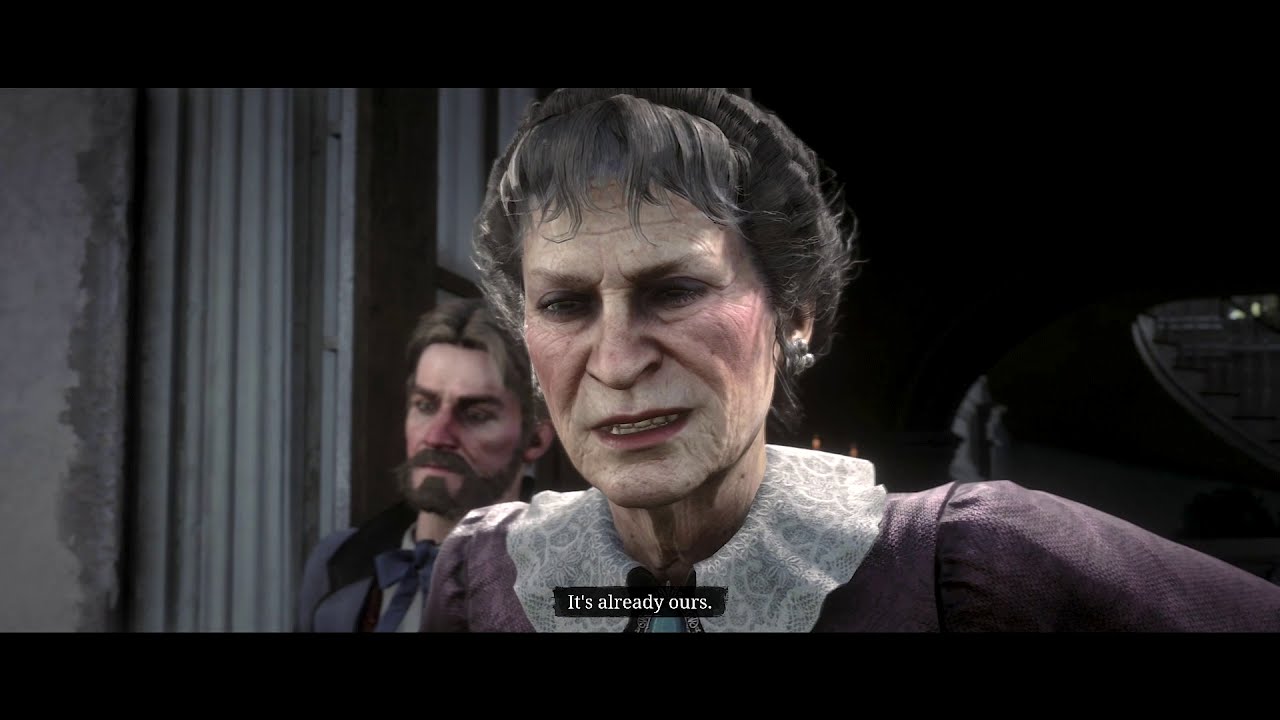The image showcases a highly realistic, digitally-created older woman, prominently featured from shoulders up, with distinct facial attributes including short charcoal-gray hair, brown eyebrows, and deep wrinkles. Her pale skin is accentuated with heavy blush and pink lips, and her mouth is slightly open, revealing her teeth. She dons a vintage outfit comprising a lacy white collar and a dark eggplant purple tweed garment. Behind her and slightly to the right, a bearded man with dark brown hair parted in the middle and a mustache looks downward, suggesting a somber mood. Both characters wear expressions hinting at frustration or anger, potentially indicating a thematic backstory. The setting includes what appear to be draperies or curtains in the background. The overall aesthetic implies a scene from a video game or a 3D animated movie about zombies or a similar horror theme. At the bottom of the image, in small white font, is the phrase "It's already ours," reinforcing the eerie and possibly apocalyptic narrative.